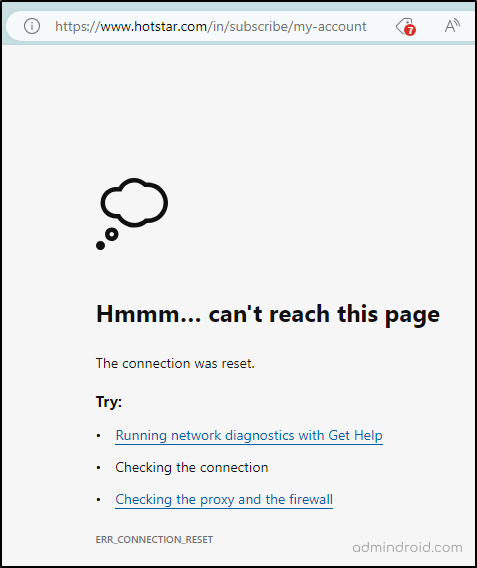**Detailed Caption:**

The image portrays a screenshot of a webpage from Hotstar.com, specifically the URL: www.hotstar.com/in/subscribe/myaccount. At the top of the page, there's an alert symbol consisting of a red circular icon with the number seven inside it. Adjacent to this is a large uppercase letter "A." To the left, there is a gray circular icon featuring a lowercase letter "i."

The search bar is situated on a background that has a greenish-gray hue. The main body of the webpage is displayed in a light gray color. Roughly halfway down the page, a cloud icon with two dots underneath signals an error message that reads: "Hmm... can't reach this page. The connection was reset."

Below the message, there's a prompt that reads: "Try the following:"

- "Running network diagnostics with Get Help," which is a clickable blue link.
- "Checking the connection," written in black text.
- "Checking the proxy and the firewall," also a clickable blue link.

Finally, at the bottom of the image, there's an error code displayed: "ERROR_CONNECTION_RESET." This suggests various steps the user can take to diagnose and resolve their connectivity issues.